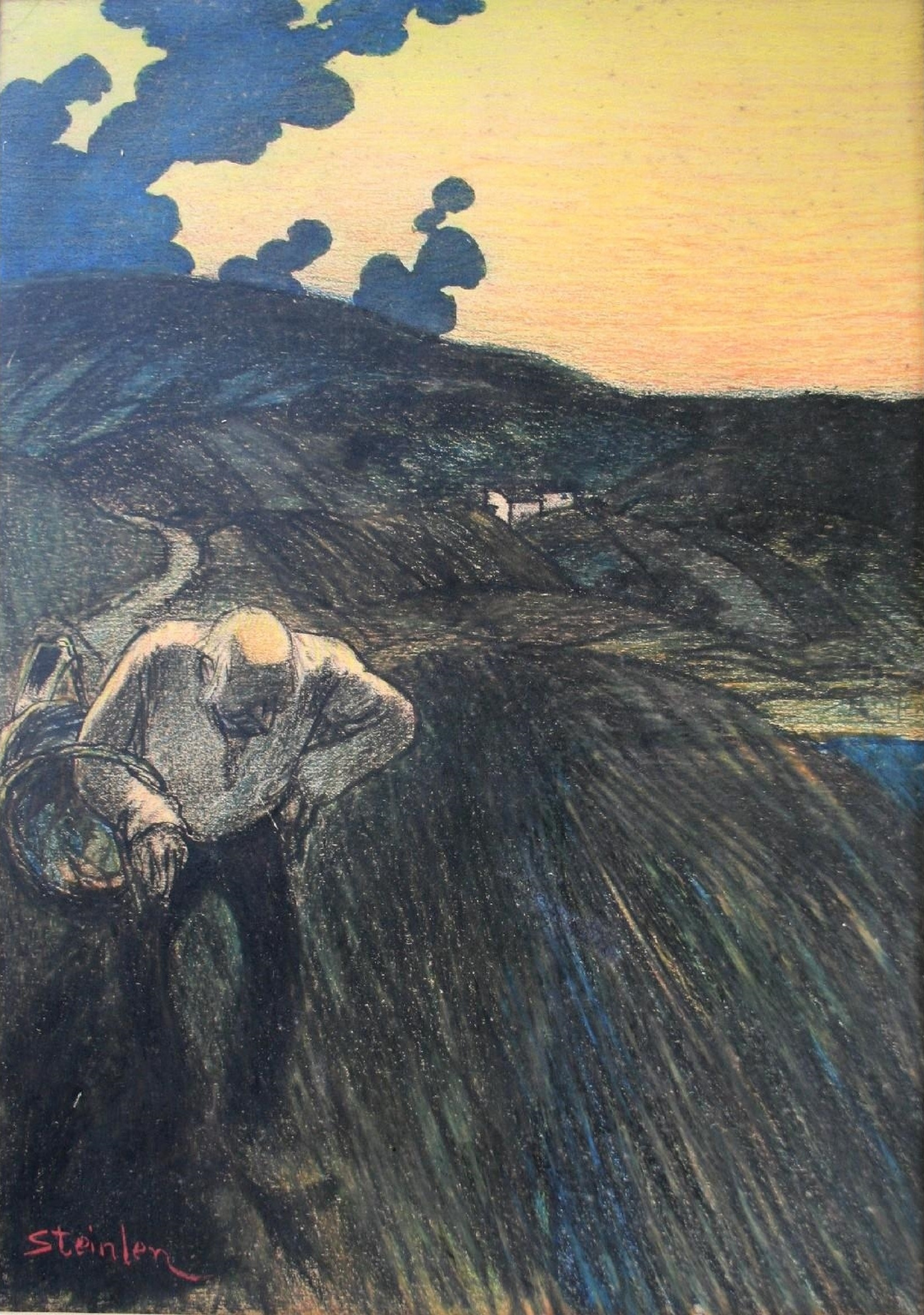This detailed pastel and charcoal drawing, titled "The Old Plowman" and created by Théophile Alexandre Steinlen around 1900, showcases a poignant rural scene rendered in a vertically rectangular portrait orientation. Dominating the lower left corner is an elderly, stooped man with a bald head framed by white hair. Dressed in a white shirt and black trousers, he carries a basket looped over his right arm. The background features a light gray trail winding through gently rolling hills, leading to small white houses nestled in the central landscape. Dark blue, black, and gold sketch marks adorn the right side, representing the land's texture. Above, dark blue storm clouds contrast with an orangish-yellow sky, adding a dramatic flair to the serene yet evocative countryside setting. The artist's red signature, "Steinlen," is prominently placed in the lower left-hand corner.